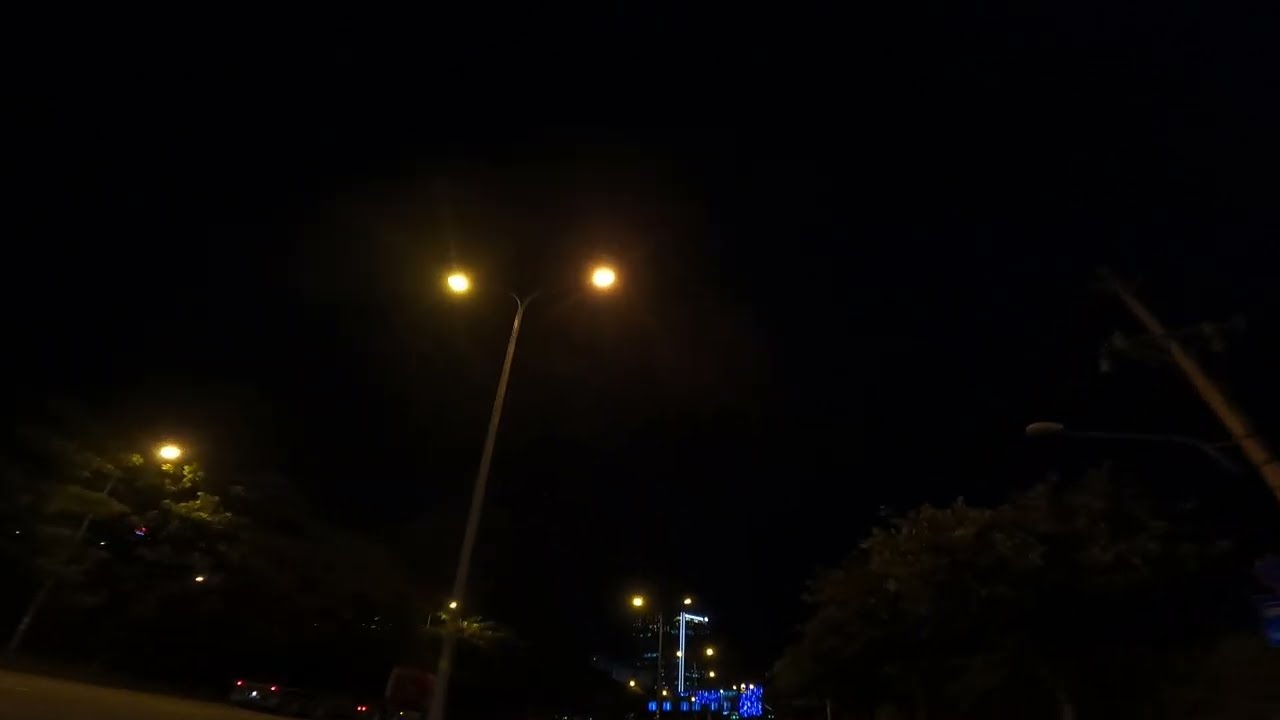The image depicts a dark, nighttime outdoor scene captured from an upward angle. Dominating the center and left portion of the horizontally aligned rectangular frame is a tall streetlight pole with two yellow lights extending in opposite directions. Just slightly left of this main streetlight, a second streetlight is partially visible amid the silhouettes of trees. The bottom of the image reveals the taillights of vehicles on a road, with faint blue road signs appearing in the center distance. The black sky fills the background, dotted sporadically with small, blurry specks of light. On the right side, another wooden pole, potentially strung with power lines and juxtaposed with additional trees, stands with its streetlight unlit. The setting is enveloped in darkness, with minimal illumination from the streetlights creating a moody urban nightscape.